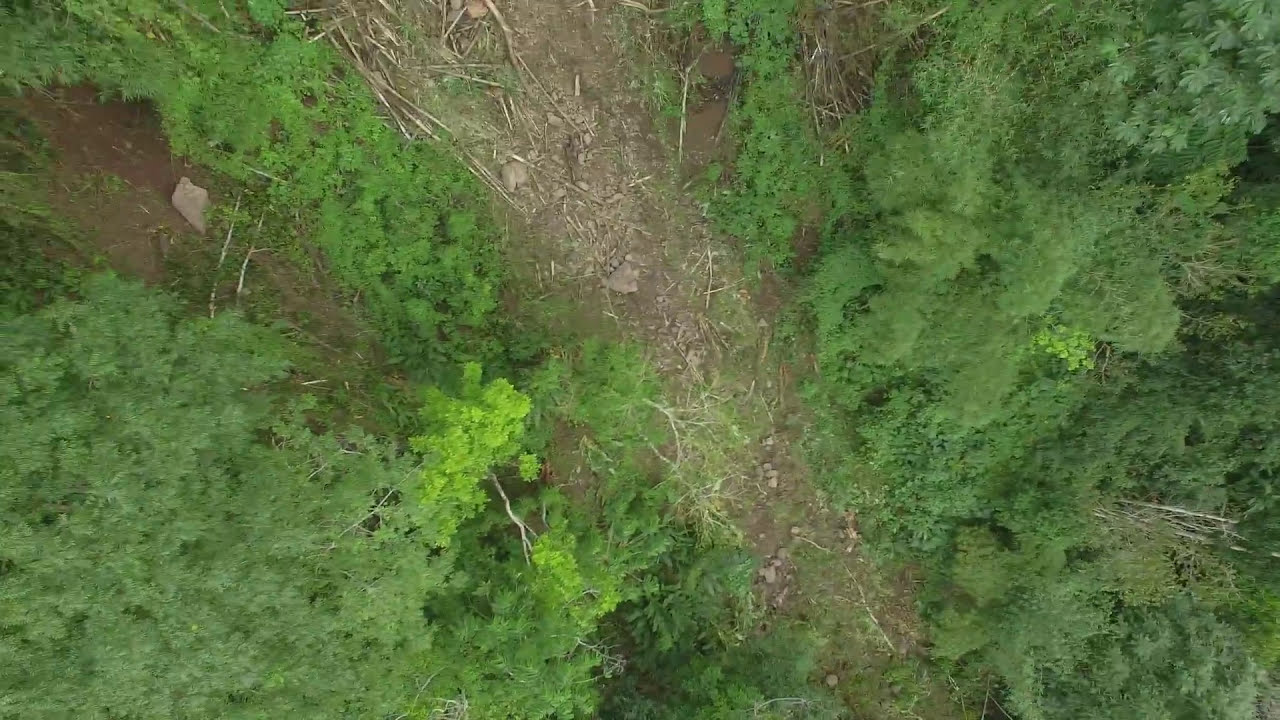This aerial photograph, captured during the daytime, showcases a densely wooded area with an abundance of greenery, including trees, shrubs, and bushes. The image prominently features a central pathway, likely a dirt or sand trail, which spans diagonally from the bottom left to the upper right of the frame. This pathway appears to be the result of a landslide, evidenced by the presence of fallen dead branches, tree trunks, and scattered debris. On the upper left corner, another smaller patch of exposed brown dirt and rocks can be seen among the green foliage. The greenery surrounding the path predominantly features medium green hues, with patches of lighter, almost yellowish-green vegetation towards the bottom left of the image. The scene is devoid of any animals, focusing solely on the natural landscape of the forest.